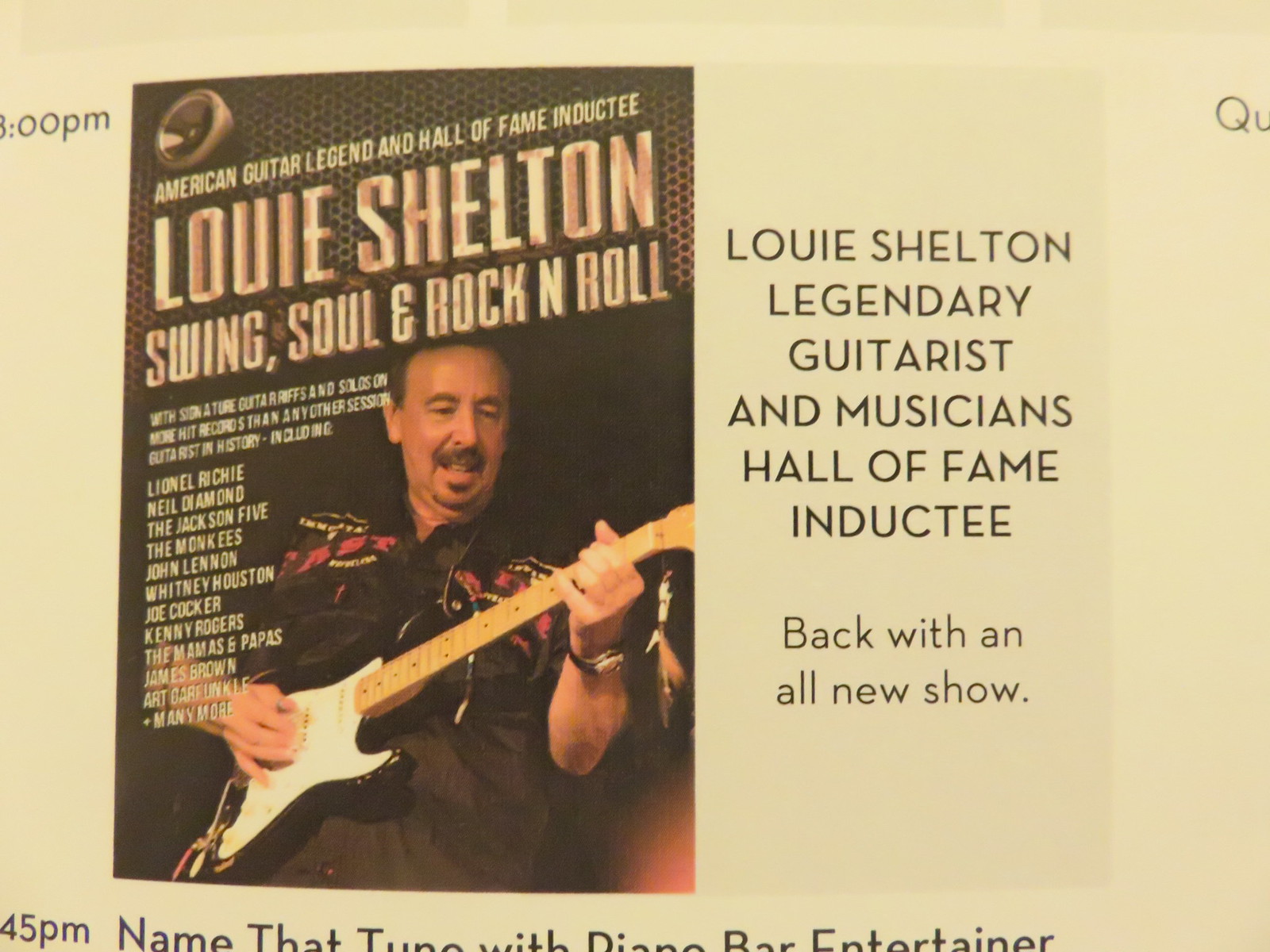This photograph captures a green-background flyer prominently featuring the legendary guitarist Louis Shelton. On the left side of the flyer is a vibrant color photo of Shelton—a white male with black hair and a mustache—leaning back while playing an old black Fender Stratocaster with a white pickguard and a light tan-colored neck. The photo, which resembles a book cover, is surrounded by white text reading: "American Guitar Legend and Hall of Fame Inductee Louis Shelton, Swing Soul and Rock and Roll." Additional, less readable white text appears beneath this section, and a vertical column with names is also present. To the right of Shelton's image, in bold black text, the flyer further emphasizes: "Louis Shelton, Legendary Guitarist and Musician's Hall of Fame Inductee. Back with an all new show." The overall appearance suggests that this is a promotional flyer or potentially a magazine cover highlighting Shelton's newest performance tour.